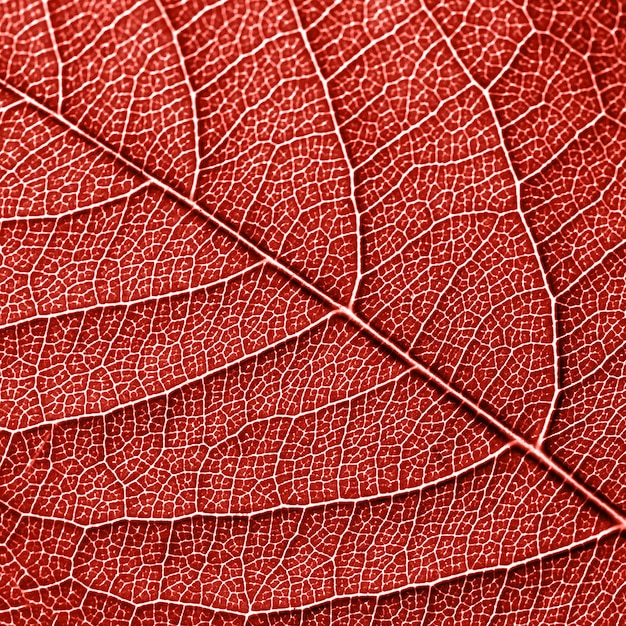This image appears to be a highly detailed, close-up view of a red leaf, captured in a manner that highlights its intricate vein structure, potentially resembling a photograph taken through a microscope or computer-generated graphic. The leaf exhibits a rich crimson or brick-red coloration, with prominent white veins creating a striking contrast against the red. The main vein runs through the middle of the leaf, slightly below the diagonal, with numerous branching veins extending from it. These veins form a complex network, connecting to each other in various patterns. Additionally, smaller veins and scaly, irregular red shapes are visible within this web-like structure. The entire image, devoid of any other elements, emphasizes the delicate, interconnected beauty of the leaf's internal architecture.